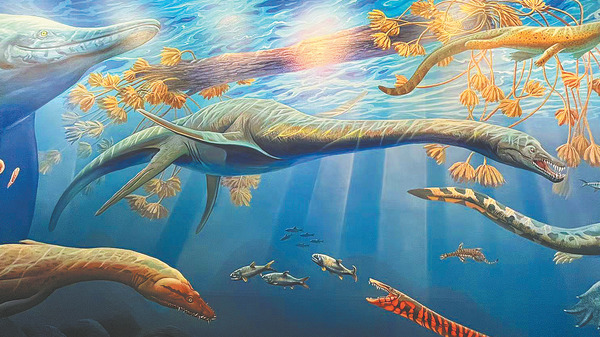This vibrant and detailed color drawing features an enchanting underwater scene with a variety of prehistoric and modern sea creatures. At the center of the image is a striking long-necked, dinosaur-like fish with an elongated, snake-like neck, an alligator-like head with an orange eye, sharp, protruding teeth, and a long, narrow tail. The creature has two short bottom fins and two side fins at the base of its neck, and it is primarily blue in color. To the bottom left, a similar reptilian fish swims, differing in its green hue.

Above this green fish is a dolphin-like creature, emerging from the upper left. It's reminiscent of a common dolphin or porpoise, adding a touch of modern marine life to the scene. The water is rendered in a bright, clear blue with shafts of light penetrating from the surface, illuminating the underwater world.

In the lower center of the image, a school of small, modern-looking gray fish swim together, being followed by another eel-like, prehistoric creature with a scale-like, orange skin and visible sharp teeth, even with its mouth closed. The backdrop includes a large, fallen tree log with drooping foliage hanging into the water, contributing to the enchanting and almost mythical atmosphere of the underwater tableau.